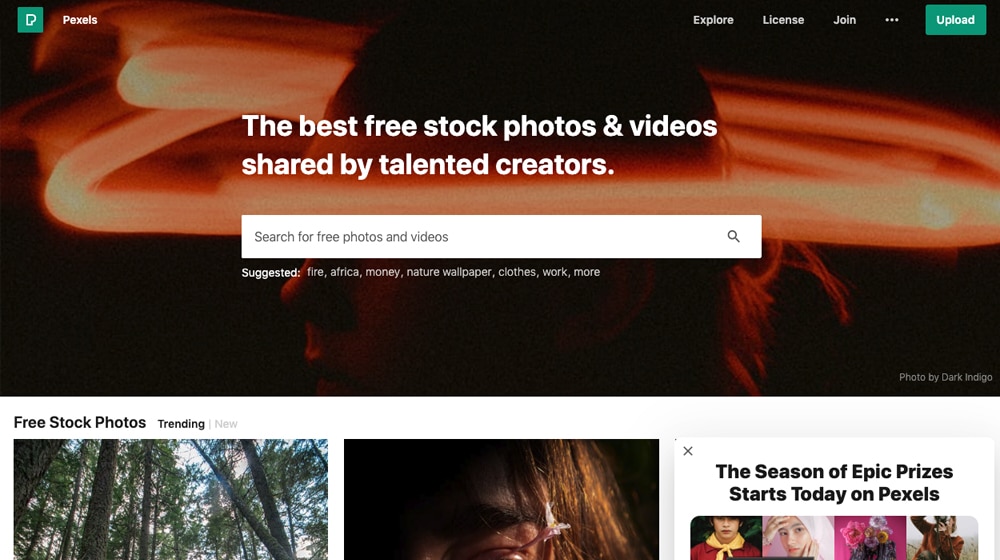This is a screenshot of the Pexels website. The top section features a modern, minimalist 'P' logo enclosed in a green square with the word 'Pexels' next to it in white text. To the right, there's a navigation menu with options labeled 'Explore,' 'License,' 'Join,' followed by three vertical dots, and a prominent green 'Upload' button. Partially visible is a blurred image of a person's head with dynamic light streaks, possibly created using a slow shutter speed technique.

The main headline reads, "The best free stock photos and videos shared by talented creators," with a search bar under this text inviting users to "Search for free photos and videos," indicated by a magnifying glass icon. Beneath the search bar, there's a list of suggested search terms: 'Fire,' 'Africa,' 'Money,' 'Nature,' 'Wallpaper,' 'Clothes,' 'Work,' and 'More.' Credit for the background image is given to 'Photo by Dark Indigo,' located at the bottom right.

Below this main section, there are three feature panels. The first panel showcases 'Free Stock Photos' with an image of trees and nature. The second, 'Trending,' appears to be a close-up of a woman's face, although the details are difficult to discern. The third panel highlights a special event with the text, "The season of epic prizes starts today on Pexels," featuring four inset images: a young boy, a young girl, some flowers, and a photographer facing the camera. The rest of the page appears cut off, so no additional details are visible.